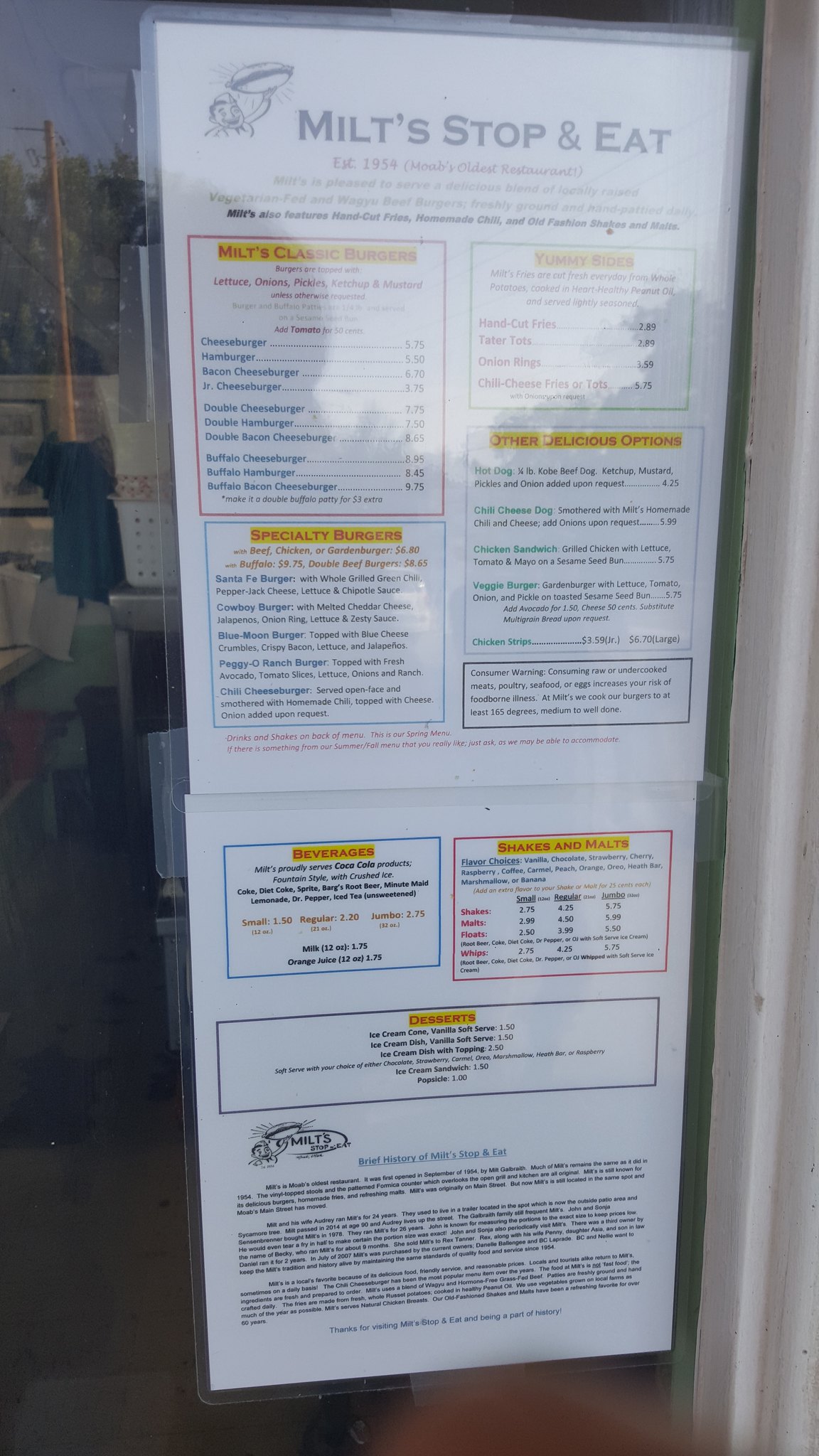This image features an outdoor menu posted on a shop window, visible through the glass. The menu, white and laminated for protection, is headed with the bold text "Melt, Stop, and Eat" at the top. Below the heading, the menu is divided into seven distinct blocks. 

The first block, a red square, contains the text "Melt [illegible] Purchase" in red lettering, highlighted with yellow for emphasis. The second, smaller square also has red text highlighted in yellow. The third block, another square, includes green details in its descriptions.

Positioned underneath these, on the right, the fourth square is labeled "Special Dangles" in red, again highlighted in yellow. The menu consists of two sheets of paper, making it appear extended. The bottom sheet has three blocks: two on the top—one blue on the left, and a red one on the right—and a longer block at the bottom with more text written at the top.

This detailed and vividly colored menu stands out against the shop's window, making it eye-catching for passersby.